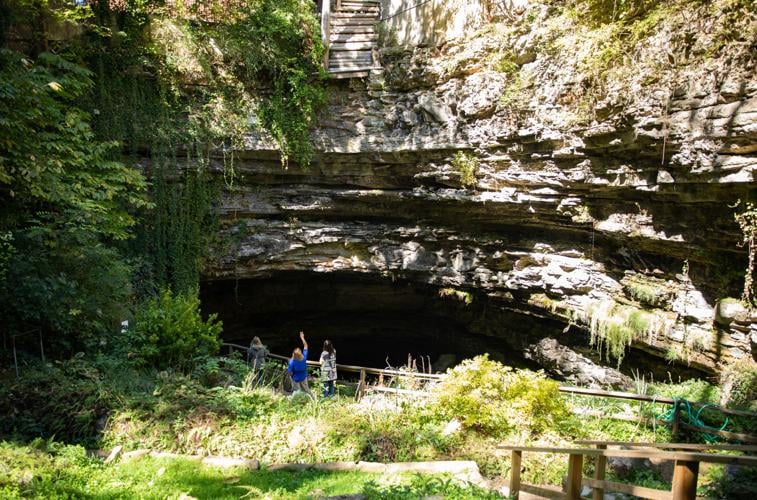The image depicts a natural outdoor scenery featuring three women standing by a wooden guardrail at the entrance of a jagged, rocky cave. Positioned on what seems to be a walking path in a park, the scene is illuminated by sunlight, highlighting the lush green grass and the abundance of trees and bushes around. The upper left of the image is filled with dense foliage and verdant greenery. The women, wearing casual attire, appear engaged with their surroundings, with one woman in a blue sweater pointing upward towards a set of broken stairs embedded at the top of the cave's entrance. The cave itself presents a dark, mysterious depth. Below the guardrail, the ground slopes downward, suggesting a possible body of water nearby, although it isn't visible in the image. Additionally, there are vine-like plants climbing the cliff's wall, and a picnic table can be spotted at the edge of the image, indicating that this area might be a popular spot for hiking and relaxation. The harmonious blend of natural elements and human curiosity captures the serene beauty and inviting mystery of the park.